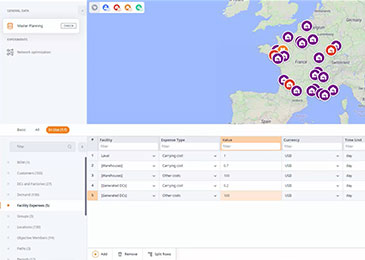A low-resolution image depicts a map of Europe with a focus on the eastern Atlantic Ocean, including Spain, France, the UK, and Germany. Numerous icons are scattered primarily around France and Germany, indicating various points of interest or data points. Unfortunately, the resolution is too low to read any text on the icons or the map itself, making it impossible to understand what the icons represent. Surrounding the map are dropdown menus and categories, which seem to offer options to modify icon appearance and highlight specific types of icons. However, due to the poor resolution, the purpose and functionality of these options remain unclear.